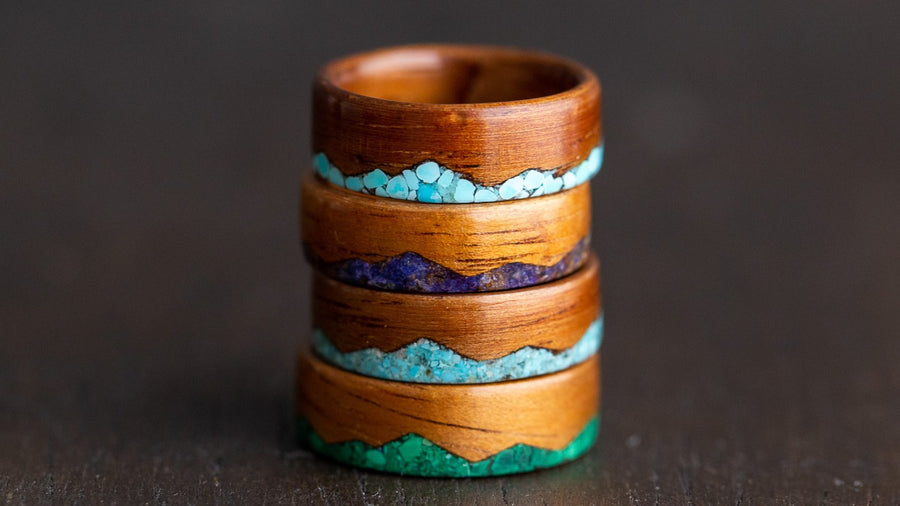The rectangular photograph, approximately six inches wide and three inches tall, showcases four wooden wristbands, or bracelets, stacked in the center on a dark brown tabletop adorned with thin black grooves. The background blurs as it ascends, highlighting the bracelets more prominently. Each wristband displays a distinguished, wavy, mountain ridge-like pattern filled with variously colored, crushed stones at the bottom.

The wristband at the top features a reddish-toned wood with large, bright blue, and white crushed stones, giving it a lustrous appearance. The second wristband from the top displays a middle blue color with a pattern reminiscent of mountainous regions, using fine, small crushed stones in deep blue and purple tones. The third wristband is crafted from lightest-colored wood adorned with a green, almost teal-like design made up of smaller rock formations, again evoking mountain ridges. The bottom wristband, similar in shape but darker green in color, incorporates larger, crushed green stones, creating a harmonious stack that captures an essence of natural, earthy textures combined with detailed craftsmanship.